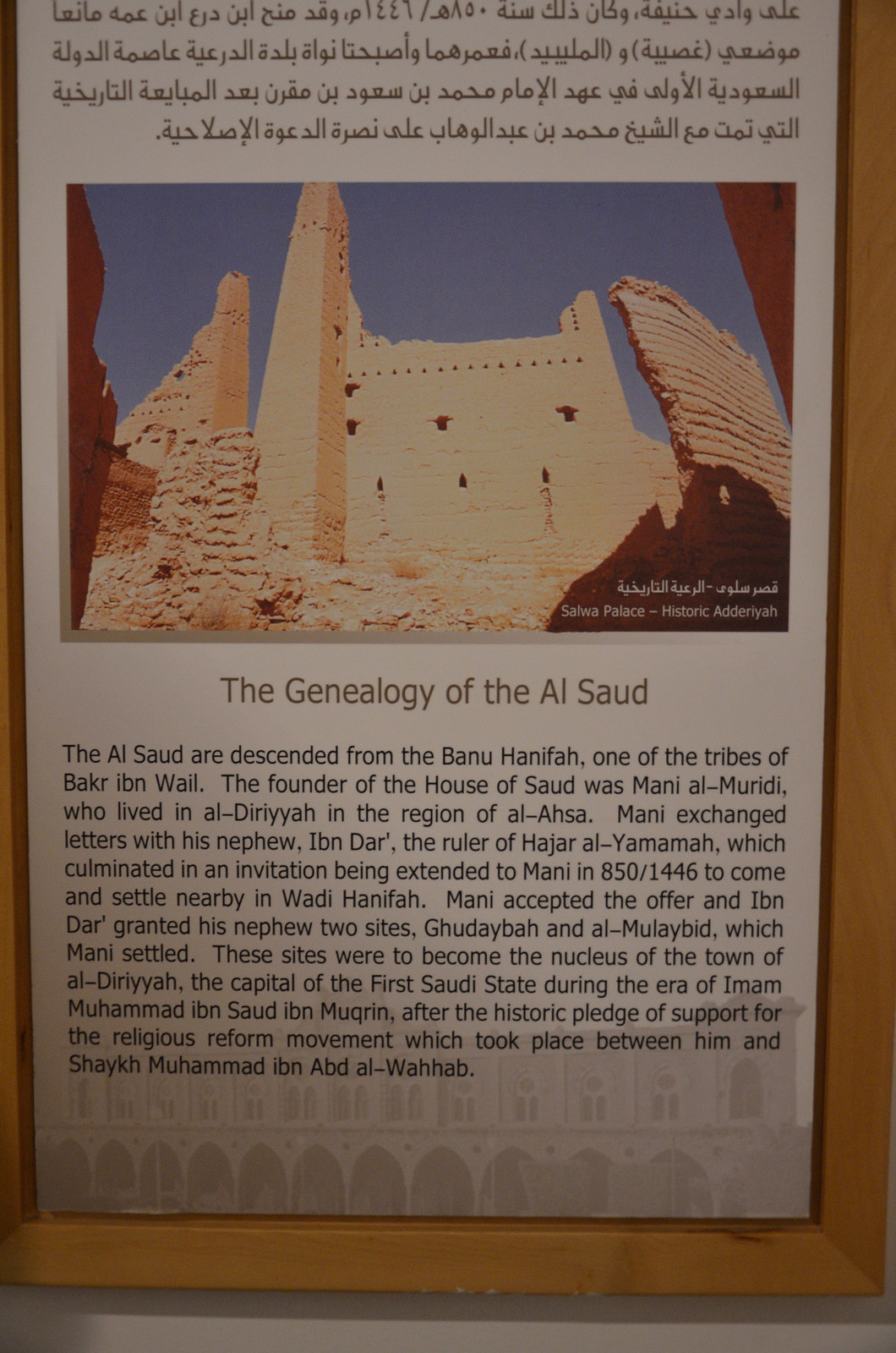The image depicts a framed photograph of an ancient building, identified as Salwa Palace, situated in a desert landscape with rock formations on either side. The frame is light brown and encloses an image featuring the decrepit palace. At the top and the right-hand side of the picture, there is Arabic writing. Below the picture, a title in beige font reads "The Genealogy of the Al-Saud." The text beneath explains that the Al-Saud are descended from the Banu Hanifa, one of the tribes of Bakr Ibn Wael. It elaborates that the founder of the House of Saud was Mani al-Muridi, who lived in Al-Diriyah in the region of Al-Asha. Mani corresponded with his nephew, Ibn Dar, the ruler of Hajar al-Yamama, culminating in an invitation extended to Mani in 850-1446 to settle in Wadi Hanifa. Accepting the offer, Mani was granted two sites, Qudaibiyah and Al-Mulaybid, which he subsequently settled. These sites became the foundation of Al-Diriyah, later the capital of the first Saudi state during the time of Imam Muhammad ibn Saud ibn Muqrin. This period marked the historical alliance between Imam Muhammad and Shaykh Muhammad ibn Abd al-Wahhab, initiating a pivotal religious reform movement.